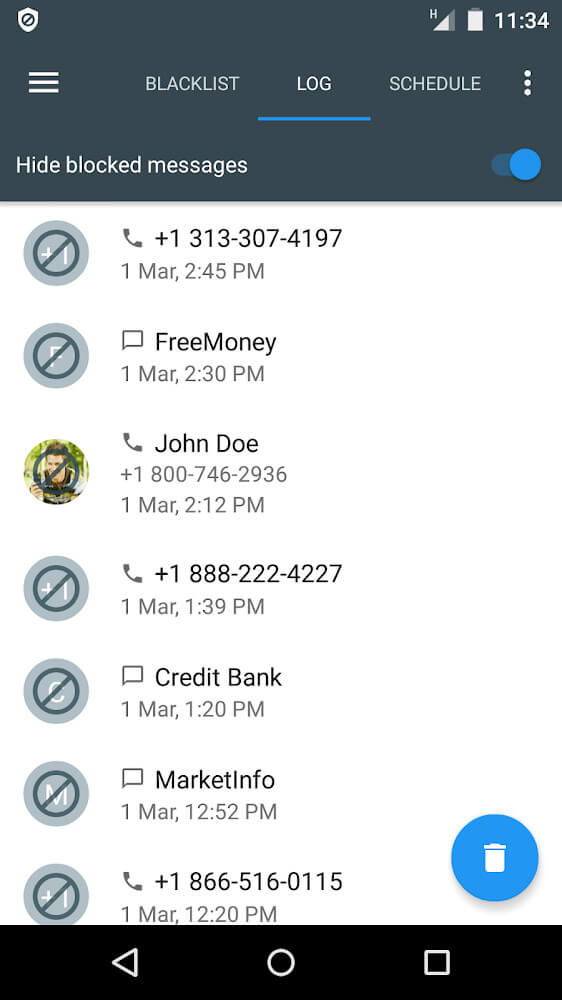This digital image is a screenshot of a phone's call log. The timestamp on the screenshot is 11:34, indicated by the clock in the status bar. In the same bar, there is a battery icon nearly full, and a Wi-Fi signal symbol showing a strong connection. 

At the top of the call log, there is an option button labeled "Hide blocked messages." Below this, the call log entries are as follows:

1. **Incoming Call**:
   - **Number**: +1 (313) 307-4197
   - **Date**: March 1st
   - **Time**: 2:45 PM

2. **Missed Call**:
   - **Identifier**: "Free Money"
   - **Date**: March 1st
   - **Time**: 2:30 PM

3. **Incoming Call**:
   - **Name**: John Doe
   - **Number**: +1 (800) 746-2936
   - **Date**: March 1st
   - **Time**: 2:12 PM

4. **Missed Call**:
   - **Number**: +1 (888) 222-4227
   - **Date**: March 1st
   - **Time**: 1:39 PM

5. **Incoming Call**:
   - **Identifier**: "Credit Bank"
   - **Date**: March 1st
   - **Time**: 1:20 PM

These entries comprise a mix of identified contacts and numbers without names, making it a detailed log of recent phone communications.